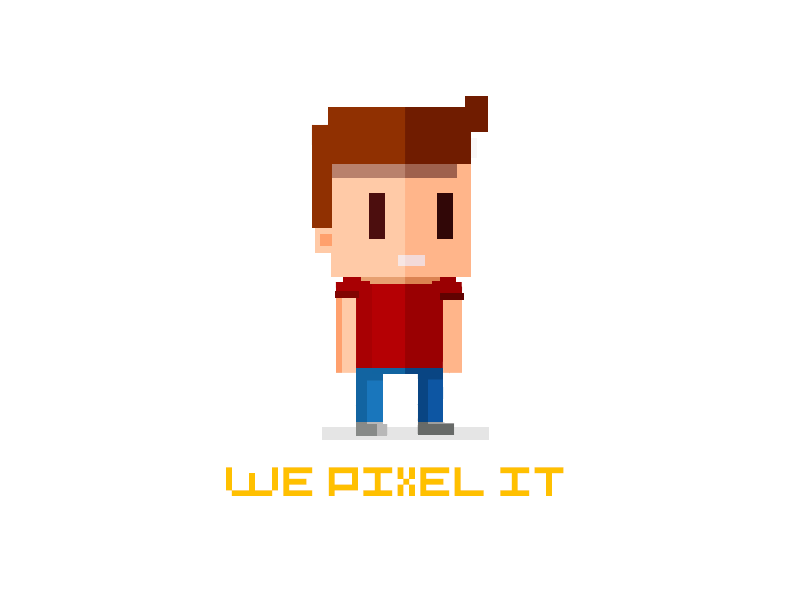This is a highly detailed pixel art image of a small, blocky character reminiscent of styles seen in games like Minecraft. The character stands against a plain white background. He appears to be a young boy with beige skin, wearing a short-sleeved reddish-brown (or red) shirt and blue pants that look like jeans. His feet are clad in small, gray shoes, and he stands on a narrow gray bar which suggests a surface. 

The boy has short brown hair with a shadow effect indicating a slight point, black, vertically-aligned eyes, and a simple white mouth. His hands rest by his sides, and there is a noticeable shading effect giving his right side a darker hue, which is due to the shadow rather than a change in skin color. At the bottom of the image, in gold uppercase letters, the caption "WE PIXEL IT" is present and also rendered in a pixelated style. The character appears endearing despite his mouth being expressionless, making him look subtly happy. The overall art style is characterized by its pixelated, geometric design.